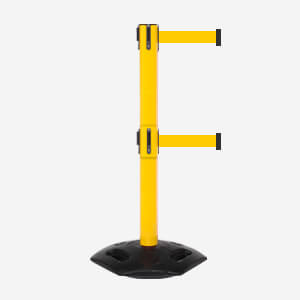The image features an object set against a soft light gray or off-white background. The central item is a yellow cylindrical pole extending vertically from a black, football-shaped base, possibly made of plastic or rubber, with four noticeable indentations or holes. Midway up the pole and at the top, two shorter yellow cylindrical bars extend horizontally to the right, creating an overall shape that resembles the letter 'F'. These horizontal bars appear to be either straps or levers, each with a black rectangular end. The device has no text, numbers, people, or animals, leading to speculation that it might be a barrier or part of a crowd control system, though its exact purpose remains unclear. The dominant colors in the image are black, yellow, and light gray.